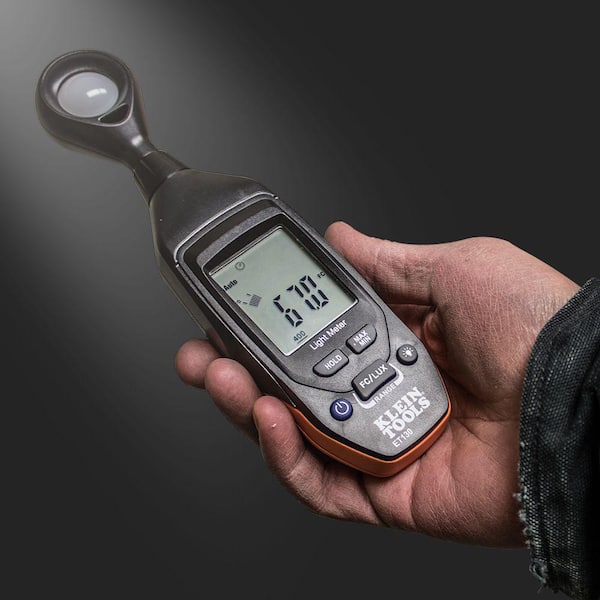The image depicts a close-up view of a rough, slightly dirty man's hand protruding from the right edge of the frame, wearing a heavy black jacket. The hand is gripping a handheld light meter from Klein Tools, model ET-130. The device, primarily black with an orange border, features a dark gray faceplate. It has a prominent circular sensor at the top, resembling a magnifying glass or an antenna, used for measuring light brightness. The center of the meter showcases an LCD screen displaying the number 67.0, likely indicating lumens or another light measurement unit. Below the screen, the text "light meter" is visible, reaffirming the tool's function. Various buttons adorn the device: a blue power button on the left, a "hold" button, a "max min" button, an "FC-LUX" button encircled by the term "range," and a black button with a light bulb icon. "Klein Tools" is printed in white letters at the bottom of the device, bringing a professional and organized look to the utilitarian gadget. The dark background emphasizes the brightness of the tool, highlighting the detailed features and robust design.